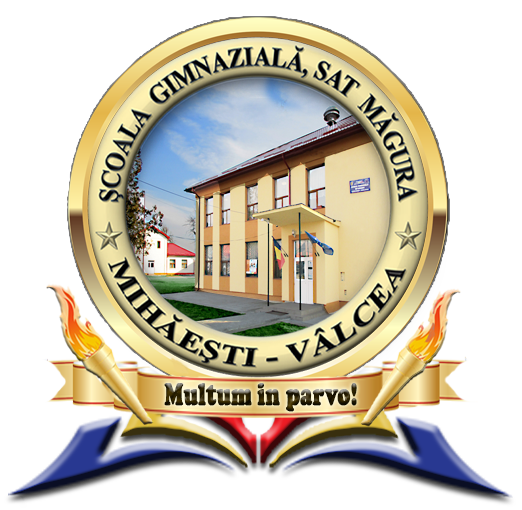The image depicts a detailed official crest or insignia set against a white background. At its center, there is a yellow, gold-textured circular emblem featuring a detailed illustration of a two-story building, resembling a municipal building, school, or town hall with numerous windows and a gray roof. The building is flanked by two torches at its base. The badge's text, written in various languages including Latin and possibly Spanish, encircles the emblem. Prominently displayed across a banner within the insignia is the Latin phrase "MOLTUM in Parvo." Below the circle, there are additional designs incorporating red, yellow, and blue accents.